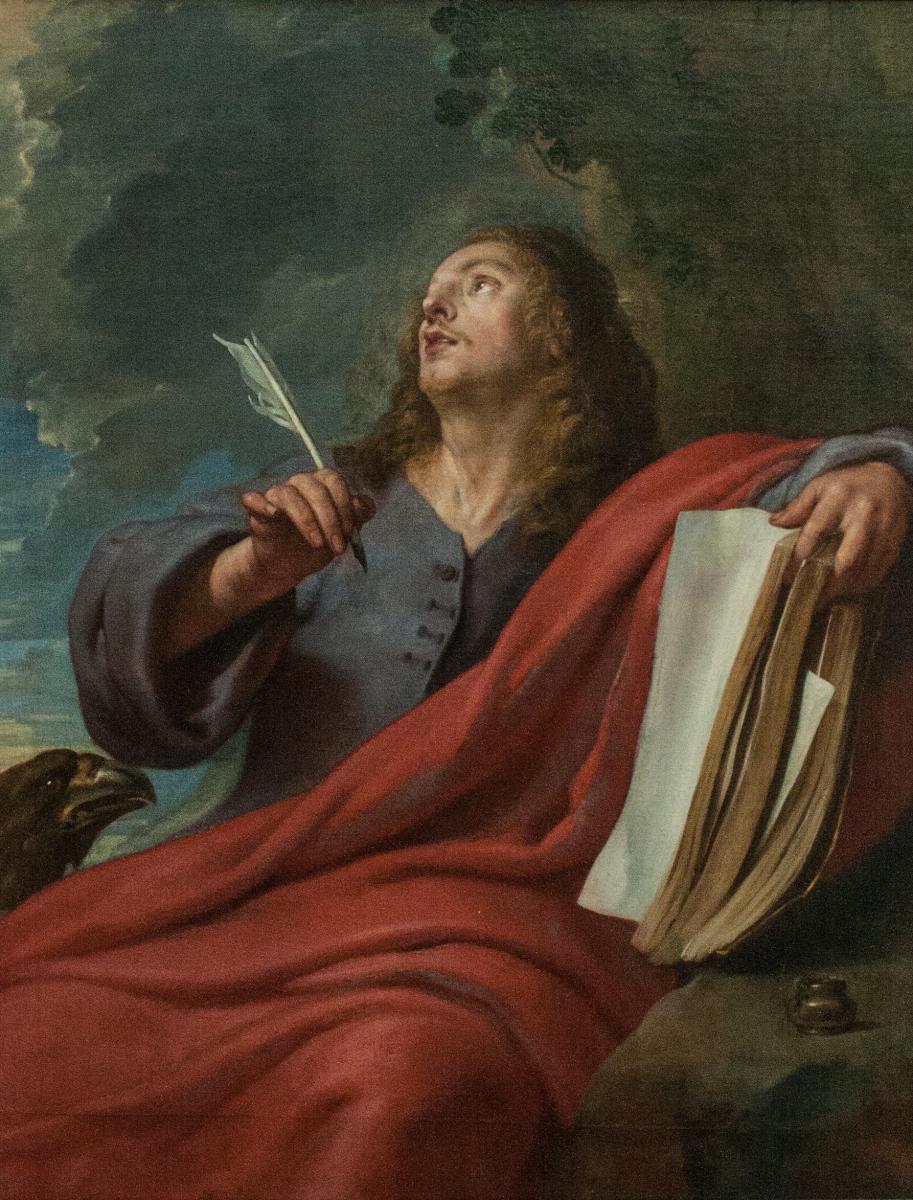The image is an intricately detailed Renaissance-style painting that captures a contemplative scene set outdoors under a cloudy sky. Dominated by muted, soft colors including shades of blue, red, green, brown, black, and beige, the artwork features a man dressed in an old-fashioned blue shirt adorned with large sleeves, partially draped in a striking red robe. Situated centrally within the composition, the man gazes upward towards the sky, seemingly deep in thought, with a feathered quill in his right hand and an open book in his left. At his feet, near a stone bench, rests an ink bottle. Adding to the serene yet solemn atmosphere, a large black bird, possibly a raven, is positioned near his right elbow. The background reveals a mix of dark and light gray clouds in the top left corner, transitioning to lighter blue skies with scattered clouds towards the middle left. A prominent tree trunk stands behind him, enhancing the natural, thoughtful ambiance of the setting.